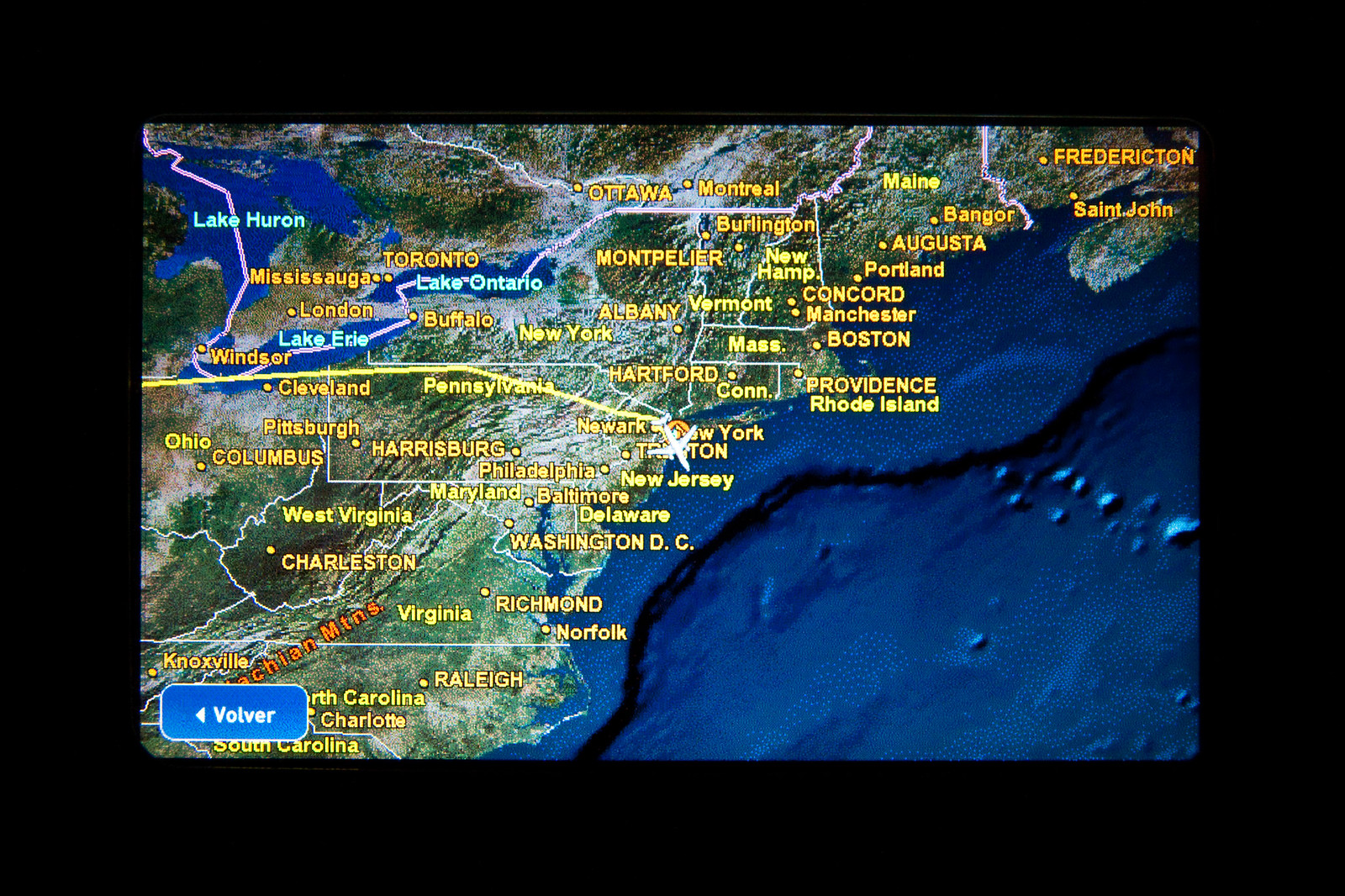This image is a detailed map of the northeastern and eastern coasts of the United States, extending into parts of the southeastern region and southern Canada. The map appears to be a satellite photograph with overlaid state outlines and yellow labels identifying various states and key cities. The whole image is framed in a black border.

On the right side, the Atlantic Ocean is visible, showcasing different depths and underwater rock formations depicted as varying shades of blue, along with a continental shelf indicating deeper waters. The landmass features intricate shading in green and white, highlighting geographical details such as jetties and bays.

The map covers a wide area, showing most of Maine with cities like Bangor, Augusta, and Portland. It extends into Canada to include parts of Quebec and Ontario, with cities like Montreal, Ottawa, Toronto, Mississauga, London, and Windsor marked. Vermont and New Hampshire are also labeled, along with New York, featuring Albany and Buffalo. Connecticut is marked with Hartford, and Pennsylvania with Philadelphia and another area mistakingly labeled as "Pennsylvania". 

New Jersey is highlighted with Trenton, and Delaware is also shown. Washington D.C. is located, with neighboring states Maryland, West Virginia (with Charleston), and parts of Ohio, including Columbus and Cleveland, making an appearance. Moving south, Virginia's Richmond and Norfolk are labeled, followed by North Carolina with Raleigh and Charlotte included. Knoxville appears under North Carolina, presumably as a labeling error. Lastly, a small section of South Carolina is visible in the bottom left corner.

Additionally, in the bottom left corner of the image, there is a blue button with curved edges that reads "Volver" (V-O-L-V-E-R), accompanied by a left-pointing triangle, suggesting a return or back function.